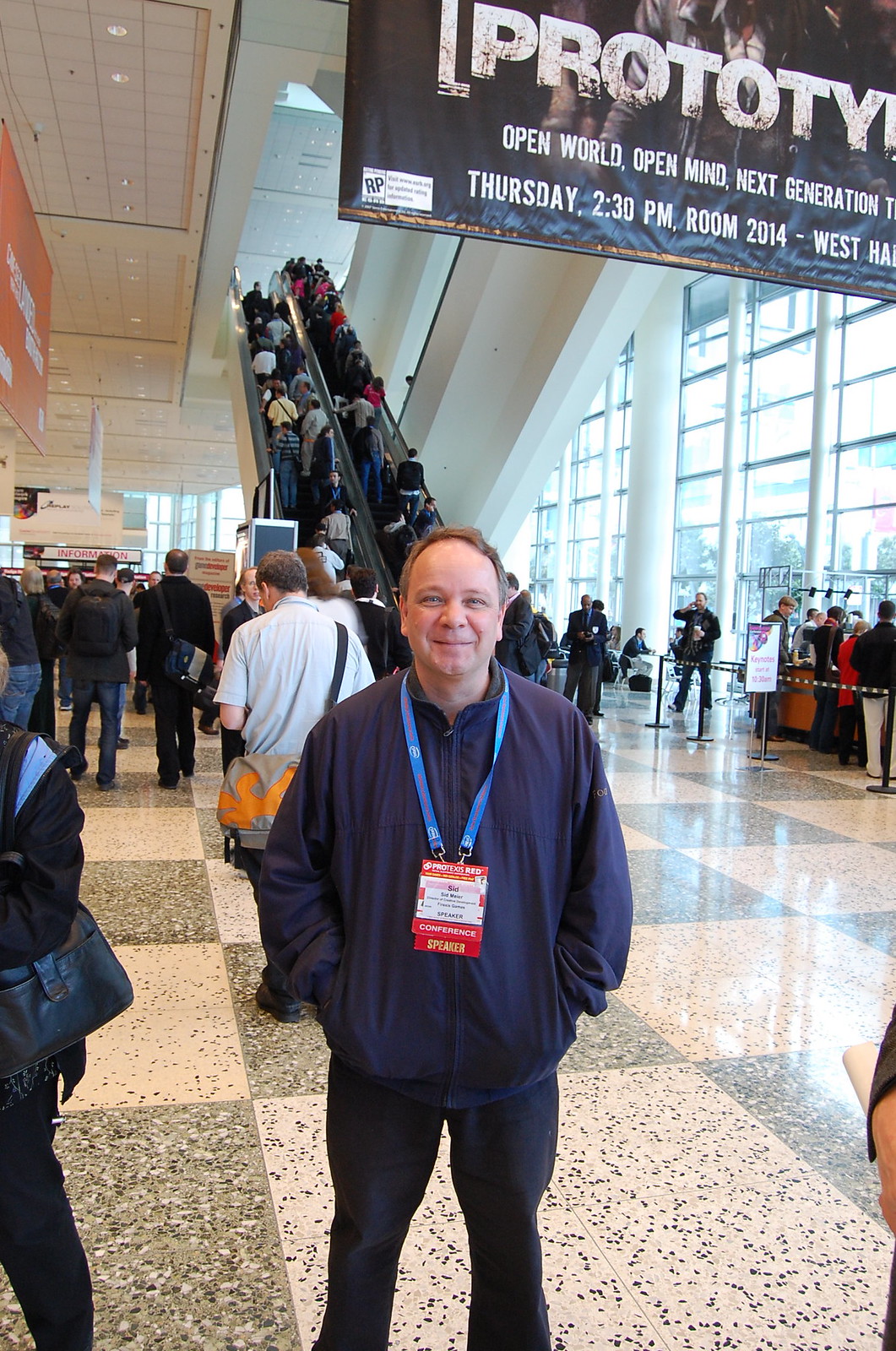In this detailed photograph, a man identified as Sid stands confidently in the middle of what appears to be a large, bustling conference or convention center. He sports a blue windbreaker or jacket, black jeans, and a visible name tag around his neck, marked "Conference Speaker" in red and white with a blue lanyard. Sid, a Caucasian man approximately five foot seven, is positioned in a well-lit lobby area in front of an escalator that is actively in use, with several people ascending and descending.

Behind him, there is a sign that prominently reads "Prototype, Open World, Open Mind, Next Generation," providing insight into the conference’s theme. The sign further details an event scheduled for Thursday at 2:30 pm in Room 2014 of the West Hall. The setting features checkered marble floors and modern architectural elements, which could place this scene inside a convention center, hotel lobby, or similar large indoor venue.

Additional individuals in the scene include a man in a white shirt with an orange and gray bag slung over his shoulder and a woman to Sid's left, identifiable only by her purse. Both are part of the buzz of activity that fills the background, adding to the atmosphere of a lively and crowded event.